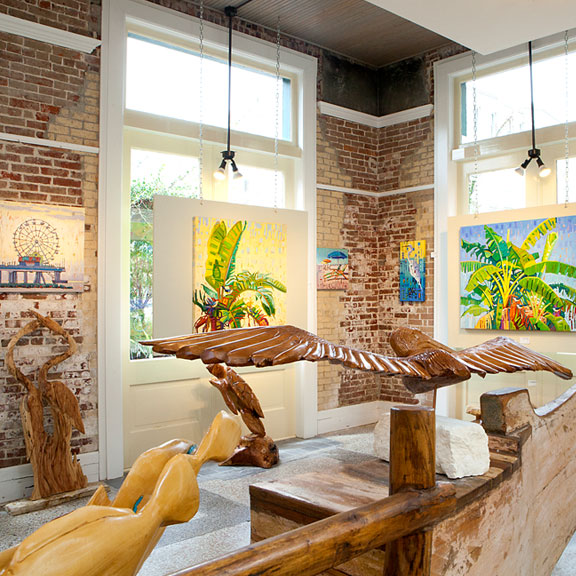The image showcases an art gallery or museum with prominent red brick walls accented by white wood trim. Central to the scene are large bay windows that flood the room with natural light. In front of each window, there are vibrant paintings of tropical banana or palm fronds in vivid greens, yellows, and blues. 

Ceiling floodlights illuminate the space, highlighting a magnificent hand-carved wooden eagle with an impressive wingspan, seemingly suspended in mid-air. Accompanying the eagle are several other hand-carved wooden sculptures, possibly including pelicans, set on polished wooden stands.

On the right side of the image, a painting of banana plants is visible, set against the backdrop of a bay window. Adjacent to this, another painting showcases a colorful beach scene with beach chairs and umbrellas, enhancing the tropical atmosphere. Above the sculptures, a painting depicting a Ferris wheel on a beach pier adds a whimsical touch to the display. To the far right, a vibrant depiction of tropical leaves and a bright sky blue background competes for attention with a striking image of a green condor against a dynamic backdrop.

The combination of detailed carvings and vivid paintings creates a rich, textured visual experience, encapsulating both natural beauty and artistic craftsmanship.